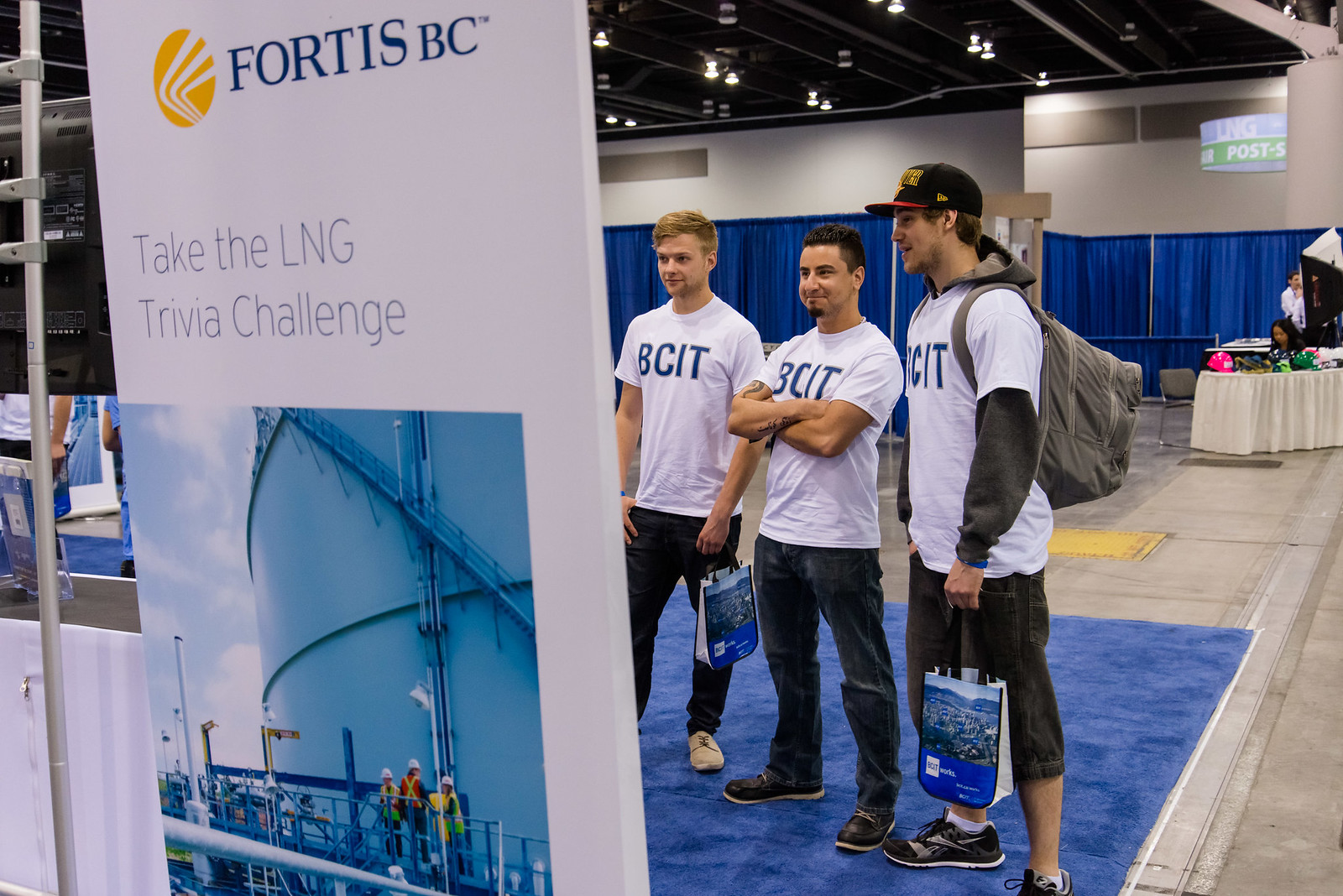The photograph captures three young men standing on a blue rectangular carpet at what appears to be a job fair or trade show inside a warehouse-like convention center. All three are wearing matching white short-sleeved t-shirts emblazoned with the initials "BCIT" in bold blue letters with a light gray outline. The young men are arranged with one in the center and two on each side, each holding tote bags adorned with blue graphics. The individual on the right is distinguishingly wearing a black baseball cap with a red brim and a large gray backpack, dressed in very long jean shorts, while the other two are in jeans and sneakers.

In the foreground to their left, a vertical white sign prominently displays the text "Fortis BC" in blue letters beside a circular yellow logo. Underneath, it reads "take the LNG trivia challenge," accompanied by a photograph featuring a large cylindrical natural gas tank with workers in high-visibility vests and hard hats standing on metal railings and scaffolding. The background setting includes blue curtains draping the walls and various other booths with tables covered in tablecloths and skirts, contributing to the bustling atmosphere of the event.